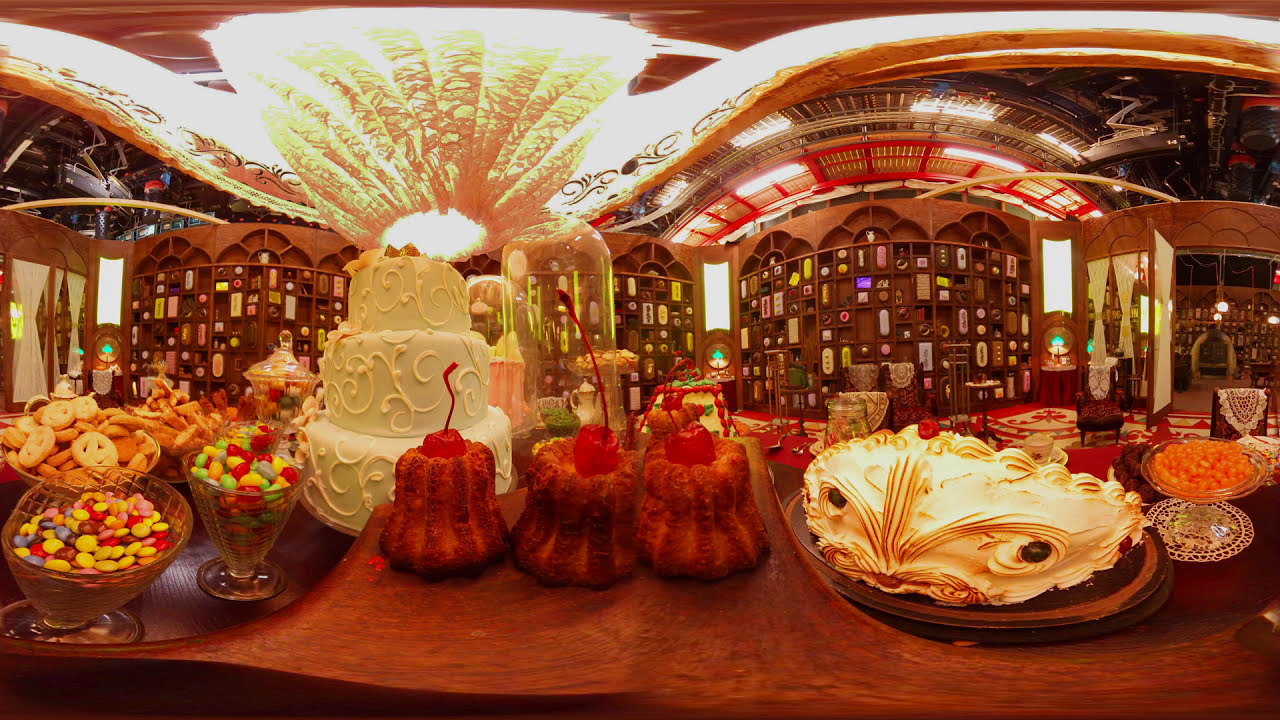The photograph captures a luxurious and elaborate indoor dessert spread, likely set in a sophisticated environment such as a hotel lobby or high-end restaurant, possibly for a celebration like a wedding. Dominating the center of the table is a three-tiered white wedding cake adorned with intricate frosting. To the left of this centerpiece, there are jars and bowls brimming with colorful candies such as M&M's and jelly beans, alongside pretzel-shaped sugar cookies. Nearby, a light blue fondant cake adds a splash of elegant color to the arrangement. On the right side, the display features three bell-shaped pastries each topped with large cherries, a slightly burnt white pie, and a whimsical cake designed to look like a dragon. Accentuating the opulent setting, brown bookcase-like structures and what appears to be signs and shelves of assorted candies enrich the background. The ceiling, with its brown and white lighting, enhances the ambiance of this grand dessert display.